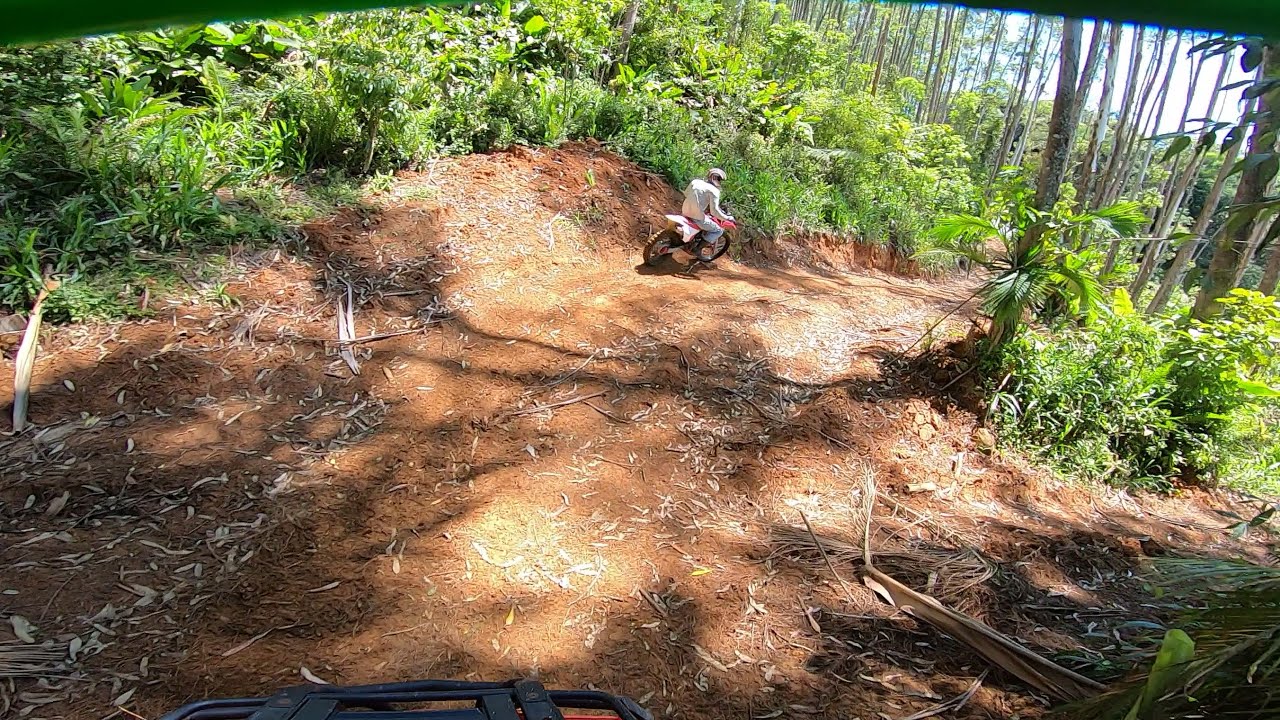This photograph captures a dirt biking trail winding through the heart of a lush jungle. The narrow, unmetalled path, composed of brown soil sprinkled with dry leaves and straw-like material, extends from the bottom of the image, converging towards the middle before turning right into the dense woodland. Along this path, a motorcyclist can be seen riding a white motorcycle, dressed in a white long-sleeve shirt, blue jeans, and a white helmet. He appears slightly off the trail but is maneuvering to get back on course. Surrounding the path, vibrant greenery dominated by alternating shades of bright green bushes and tall trees frames the scene. To the right, thick woods with tall plants and tree trunks rise, while the left side reveals more cleared areas sporadically covered with straw. At the bottom of the image, parts of a black metallic structure, likely from another bike, are faintly visible, enhancing the adventurous ambiance of the jungle setting.